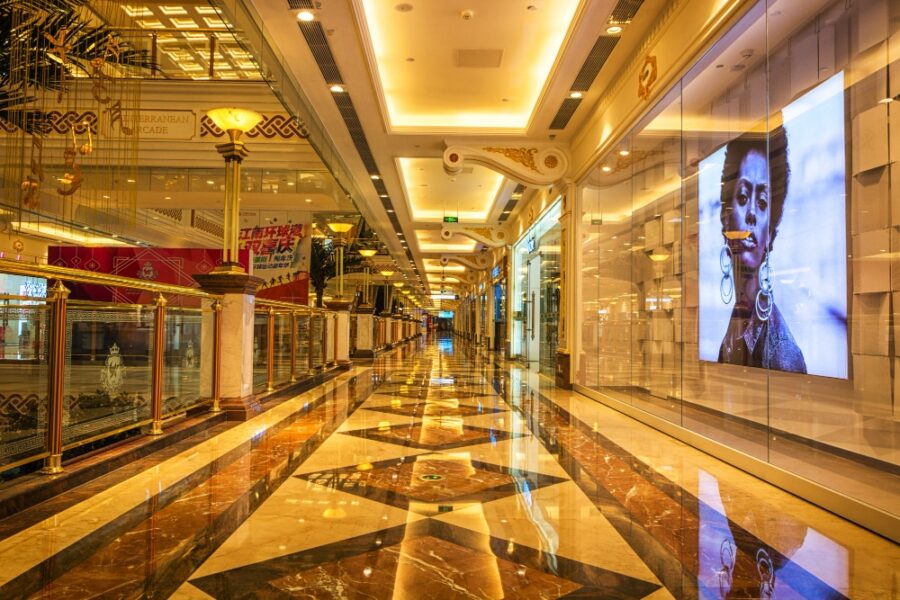This image captures a luxurious hallway, likely within a high-end mall or upscale restaurant. The walkway is characterized by a glossy, marble-style floor with an intricate design. The flooring features two long brown stripes running parallel down the hallway, each bordered by darker brown lines. In the center, light brown tiles are neatly accentuated with darker brown square outlines. The highly polished surface of the floor produces striking reflections from the ceiling lights, adding to the opulent atmosphere.

To the right, large glass windows display advertisements, including a striking image of a woman with her head slightly tilted, adorned with hoop earrings and facing the camera. This suggests commercial spaces or stores with fashionable displays. On the left, a sophisticated glass barrier spans the length of the hallway, separated by ornate brown posts with gold-tipped tops and bottoms, and topped with a gilded handrail. These posts also feature etched emblems, adding an artistic touch to the barrier.

The ceiling above is light beige, embellished with gold accents and recessed lighting framed in rectangles, enhancing the elegance of the space. Near the left side, a tall white column with brown trimmings stands out, accompanied by a long, vertical golden light fixture, contributing to the grandeur of the setting. Overall, the scene is visually dazzling and richly decorated, offering a taste of modern luxury and refined design.